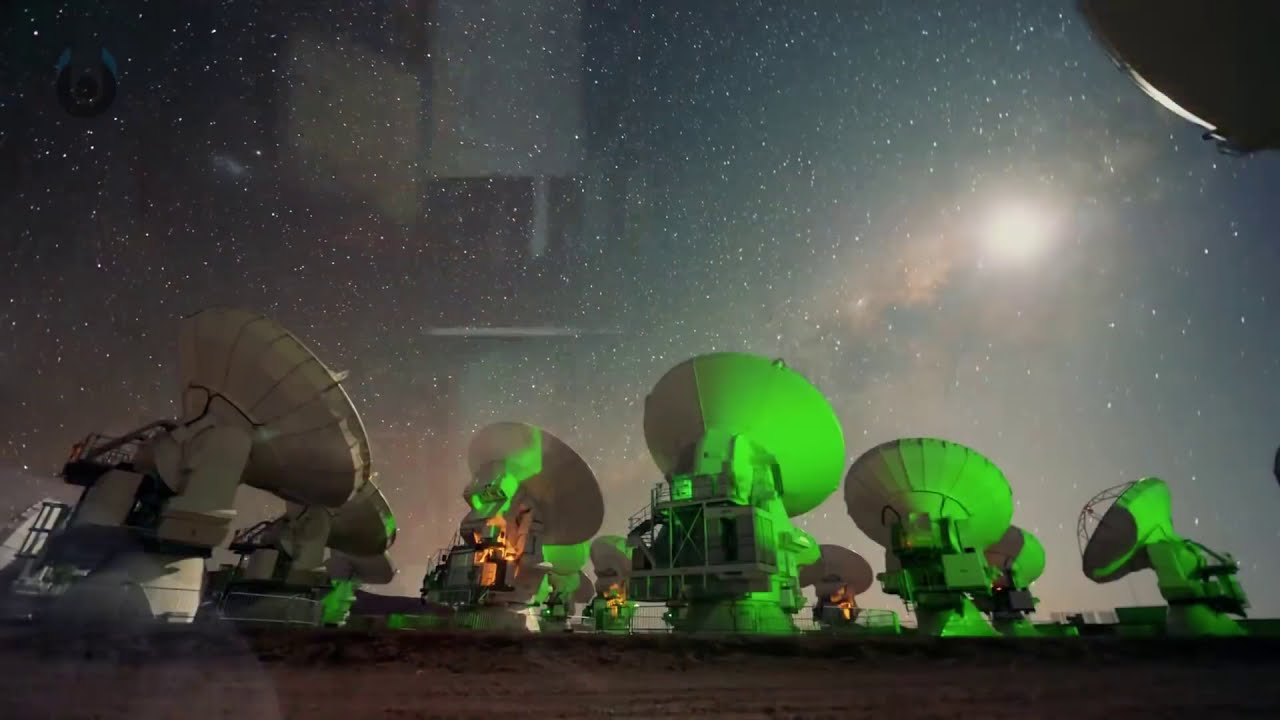The photograph features an array of space telescopes, resembling satellite dishes, all directed towards the star-studded night sky. There are nine to fifteen telescopes visible, clustered together and varying in orientation. Most of the dishes have an off-white color, with some bathed in a greenish illumination, particularly those on the right-hand side of the image. The scene is likely observed through a window, as evidenced by faint reflections and possibly a watermark in the upper left corner. The sky above is exceptionally clear and filled with stars, accentuated by a notably bright, possibly galaxy-like formation surrounded by a red, gaseous cloud in the upper right part of the image. This setup suggests the telescopes are situated far from urban lights, possibly on a high-altitude location such as Chile or Hawaii, providing an unobstructed view of deep space. The mysterious reflections on the glass add an intriguing layer to this already captivating photograph.